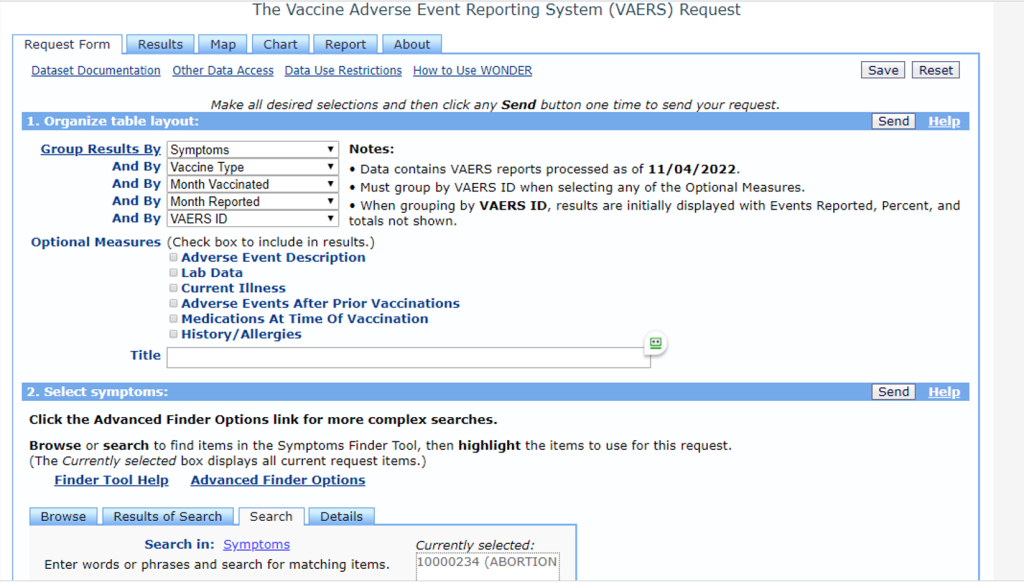This is a detailed screenshot of a website featuring the Vaccine Adverse Event Reporting System (VAERS) request interface. The webpage is set against a white background with a prominent, thick light gray vertical bar situated on its right side. At the top of the page, a thin light gray line runs horizontally across the entire width of the screen. Beneath this line, centered blue text reads "The Vaccine Adverse Event Reporting System (VAERS) Request."

The main section of the webpage starts with a navigation menu composed of tabs. The leftmost tab is white with a light blue outline, and the five tabs to its right showcase a blue gradient effect, transitioning from lighter at the top to darker at the bottom. The text on these tabs is black and they are all outlined in light blue. The tab labels are as follows: "Request Form" (the selected tab), followed by "Results," "Map," "Chart," "Report," and "About."

The content area below the tabs is enclosed in a medium-width blue outline. In the top left portion of this content area, there are links written in underlined blue text: "Data Set Documentation," "Other Data Access," "Data Use Restrictions," and "How to Use WONDER" (with "WONDER" in all caps). In the top right corner, two gray buttons with darker gray outlines and black text are labeled "Save" and "Reset" respectively.

Centrally positioned below these buttons, a small italicized line of black text reads, "Make all desired selections and then click any Send button one time to send your request." The word "Send" is bolded for emphasis.

Further down, a light blue header with white text displays the title "WONDER." On the left side of this header, it states, "Organize Table Layout:".